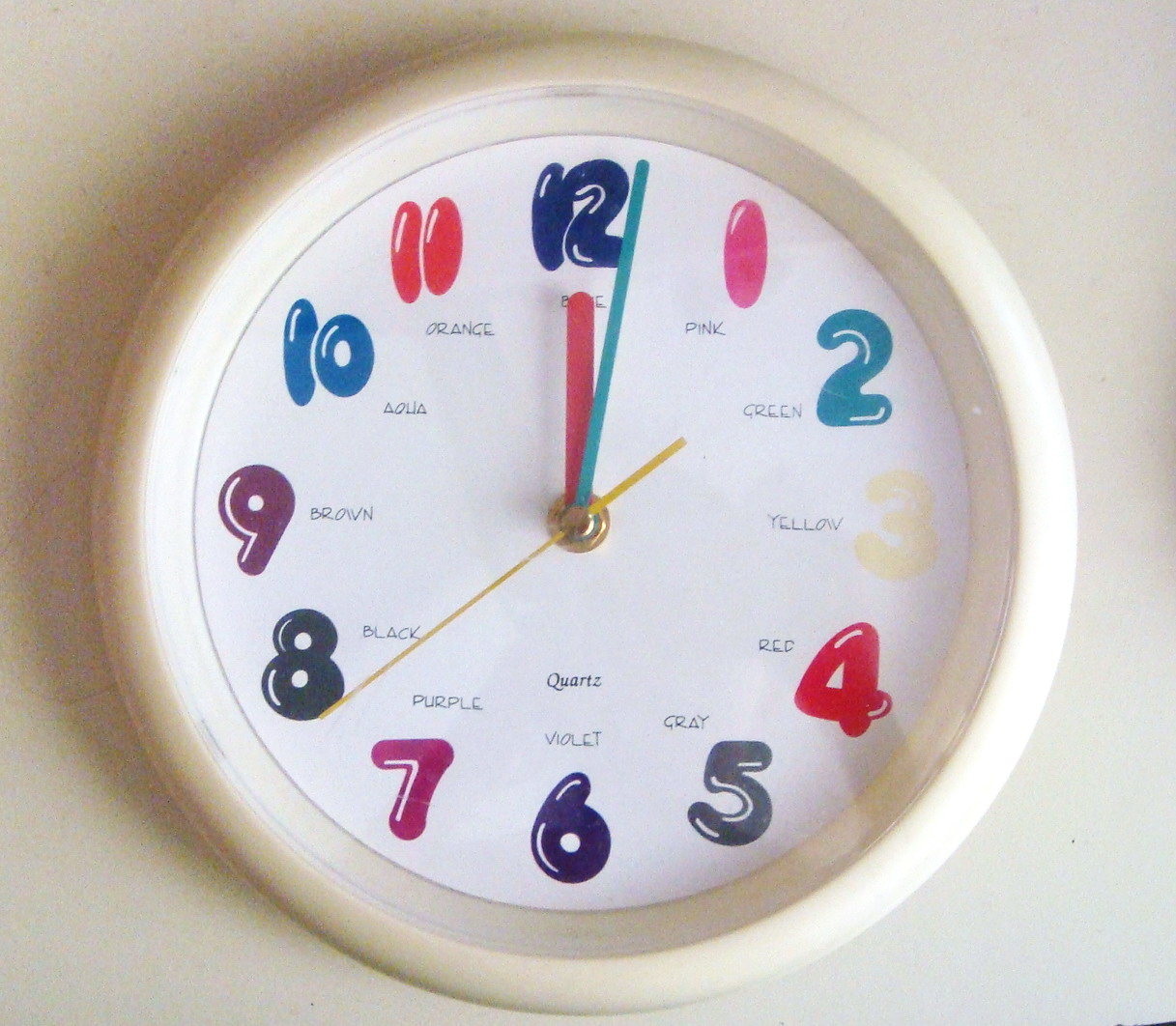This photograph depicts a close-up view of a white, round child's clock, set against a white background. The clock features bubble-letter numbers that are distinctly colored and labeled with their respective color words: a blue 12, a pink 1, a green 2, a yellow 3, a red 4, a gray 5, a violet 6, a purple 7, a black 8, a brown 9, an aqua 10, and an orange 11. The clock also has three hands: a short red hour hand pointing at the 12, a longer light blue minute hand just past the 12, and a thin yellow second hand situated between the 7 and 8. The white plastic body and frame emphasize its vibrant and educational design, intended to help children associate colors with numbers.